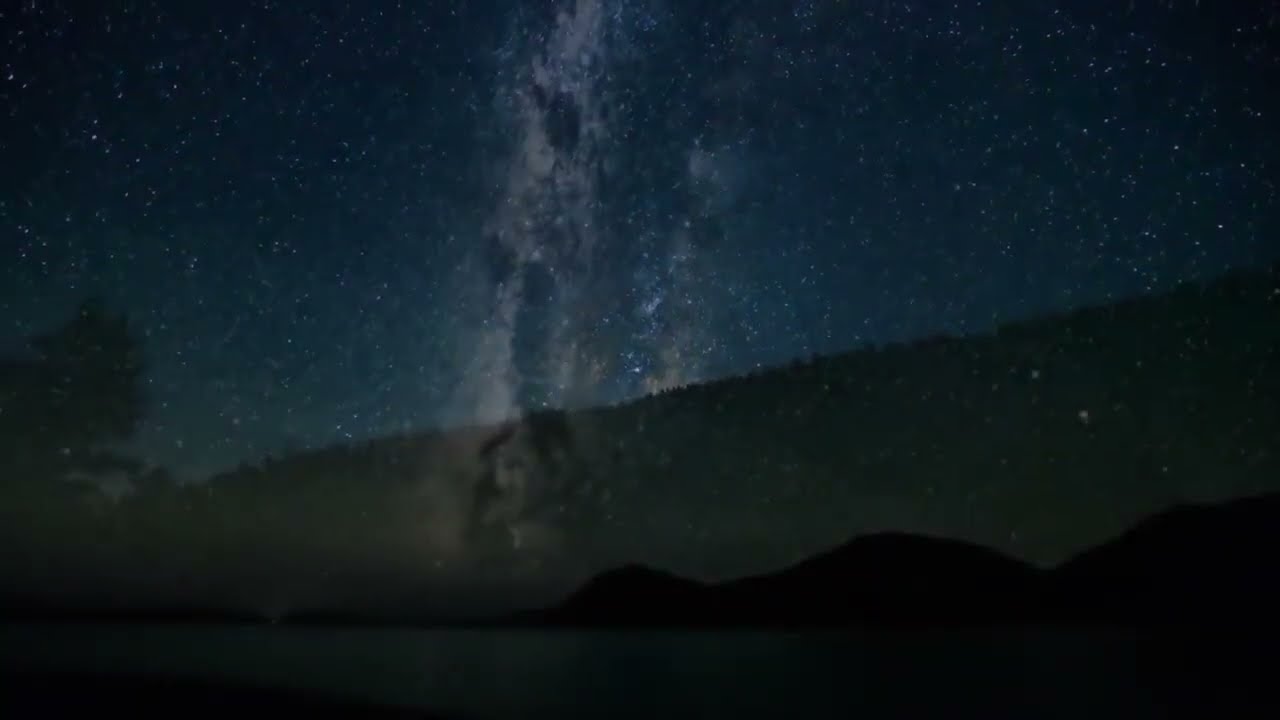This is a photograph taken at night of a dark, grassy mountainside with multiple hills forming a clustered landscape. The dark navy sky forms the backdrop, dotted with faint stars, giving the sense of a night-time setting. The mountainous terrain appears to stretch from the left, rising towards the right, with one notably taller hill featuring three distinct humps. On the far left side of the image, there is a tall tree. In the center of the image, a mysterious white mark stands out, resembling either a light or a burn mark. The overall image looks as if it might be superimposed with another, creating a surreal effect that hints at the Milky Way or a face-like figure on the hillside, making the scene intriguing yet difficult to fully discern.